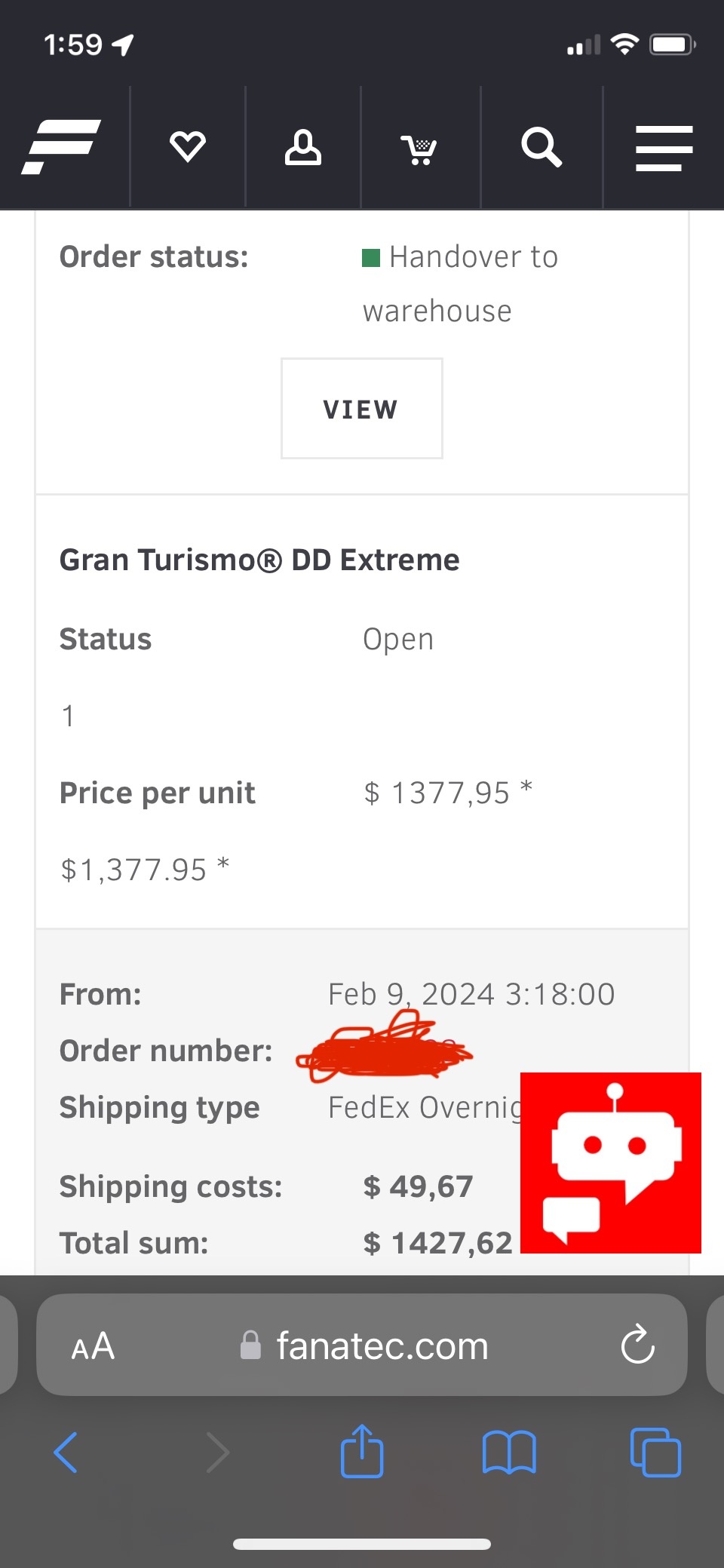This screenshot from a cell phone display captures several interface elements and details about an order status. The phone's black header at the top shows the time "1:59" in white text on the upper left, followed by a logo resembling an uppercase "F" in white. To the right of this logo, there are four icons: a white heart, a person, a shopping cart, and a magnifying glass. At the top right corner, the status indicators show two out of four bars of reception, Wi-Fi enabled, and a fully charged battery.

Below the header, against a white background, is a section labeled "Order Status." Beneath this label, the update "Hand over to warehouse" is shown, coupled with a button labeled "View." Directly below, in bold black text, is the product name "Gran Turismo DD Extreme." The status of this item is marked as "Open." The price per unit is listed as $1,377.95, with a date stamp indicating February 9, 2024, and a reference number "318" at the end.